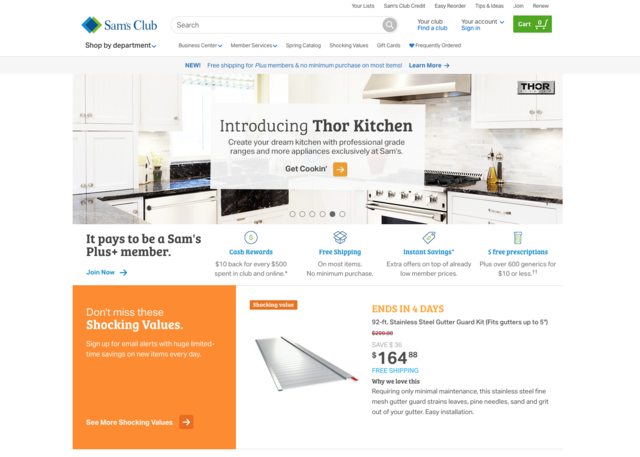The image showcases the homepage of the Sam's Club website, prominently featuring the brand's icon and name in the top left corner. Centrally placed along the top is a search bar, while a green cart button is positioned on the top right. Dominating the header is an advertisement for Thor Kitchen, highlighting the tagline: "Introducing Thor Kitchen. Create your own dream kitchen with professional grade ranges and more appliances exclusively at Sam's." This section also includes an inviting orange button labeled "Get Cookin'."

Beneath the header, a section details the benefits of Sam's Club membership, using blue icons and text for emphasis. These benefits include "Cash Rewards," "Free Shipping," "Instant Savings," and "Three Free Prescriptions," each illustrated with respective icons: a pill bottle, a dollar sign tag, an open box, and a coin with a money symbol.

Further down, the page is divided into two distinct sections. On the left, a large orange square grabs attention with the message, "Don't Miss Shocking Values." To the right, an advertisement showcases a 92-foot stainless steel gutter guard kit priced at $164.88, accompanied by an orange urgency notification noting that the offer ends in four days.